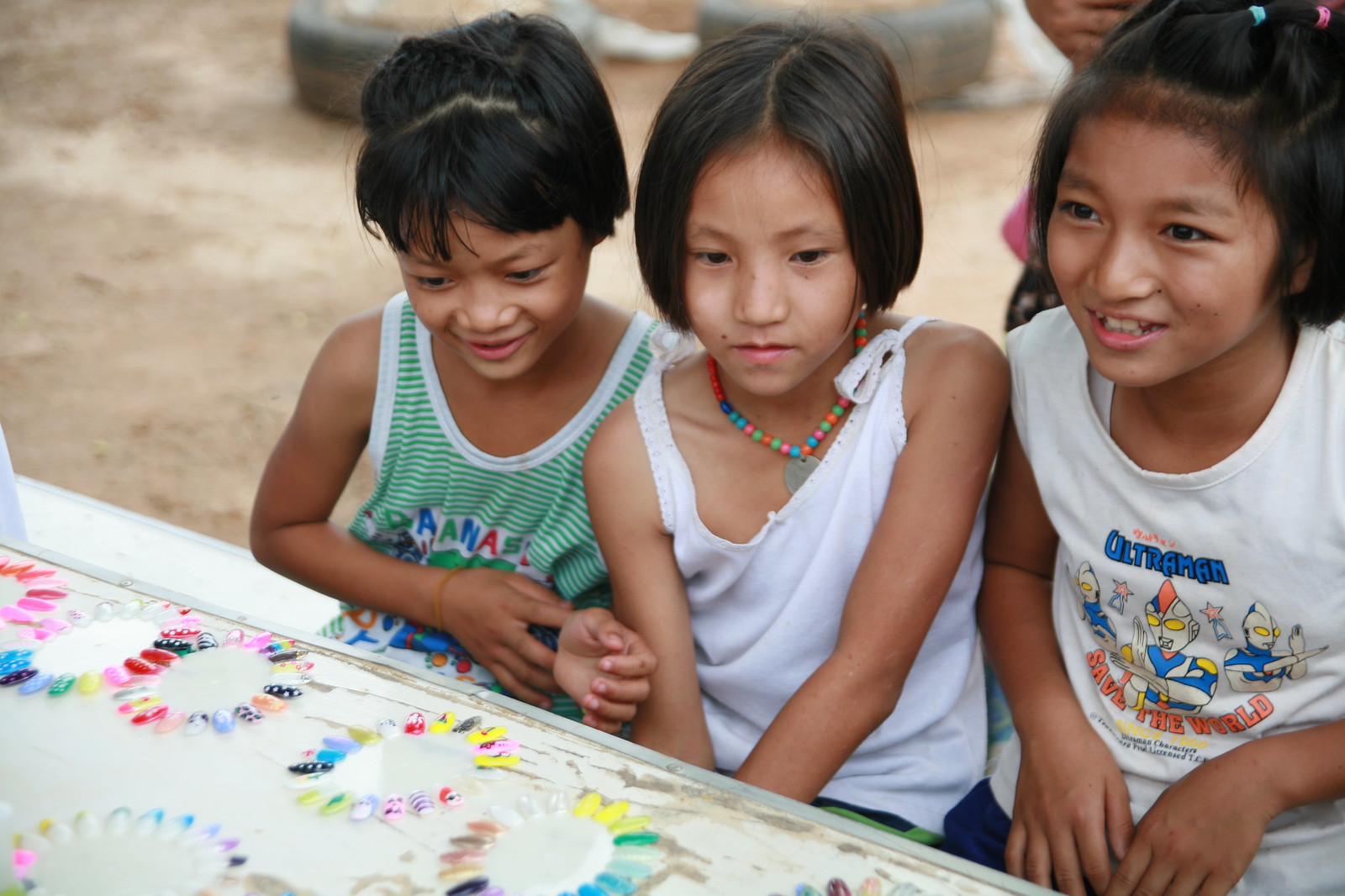In this image, three little girls with black hair are sitting side-by-side on a bench at a table, centered in the photo. The girls are wearing sleeveless shirts – the one on the left sports a green striped tank top, the middle girl wears a white tank top, and the girl on the right has a t-shirt with an Ultraman saves the world graphic. They all appear happy, with two of them smiling broadly and the third showing a subtler smile. In front of them on the table, decorative fingernail designs are laid out in little circles, suggesting they might be excited about getting their nails done. The surroundings suggest an outdoor setting in a possibly third-world or Southeast Asian community, with a sandy or dirt ground and tires visible in the background. It's daytime, and the scene is vibrant with colors like white, red, pink, purple, light blue, green, yellow, brown, and tan.